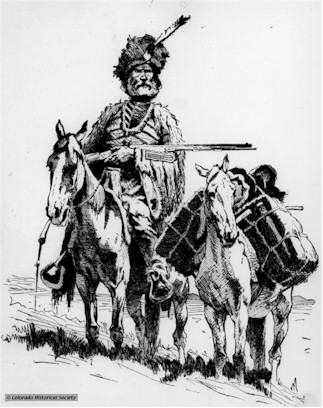This striking black-and-white image, reminiscent of a hand-drawn painting, prominently features an older, bearded American Indian man seated on a horse, evoking the stoicism and ruggedness of an old Western character. He wears a hat adorned with a feather, possibly resembling a turban, and is draped in animal cloaks, further emphasizing his traditional attire. In his hand, he firmly grasps a rifle. Beside him stands a second, smaller horse, burdened with pack gear, possibly containing a sleeping bag. The setting appears to be an expansive, flat, grassy plain, though the background remains starkly white, drawing full attention to the central figures. In the bottom left-hand corner, the image is marked with the text "Colorado Historical Society," serving as a watermark. This intricate scene encapsulates a moment of solitude and resilience, steeped in historical and cultural significance.